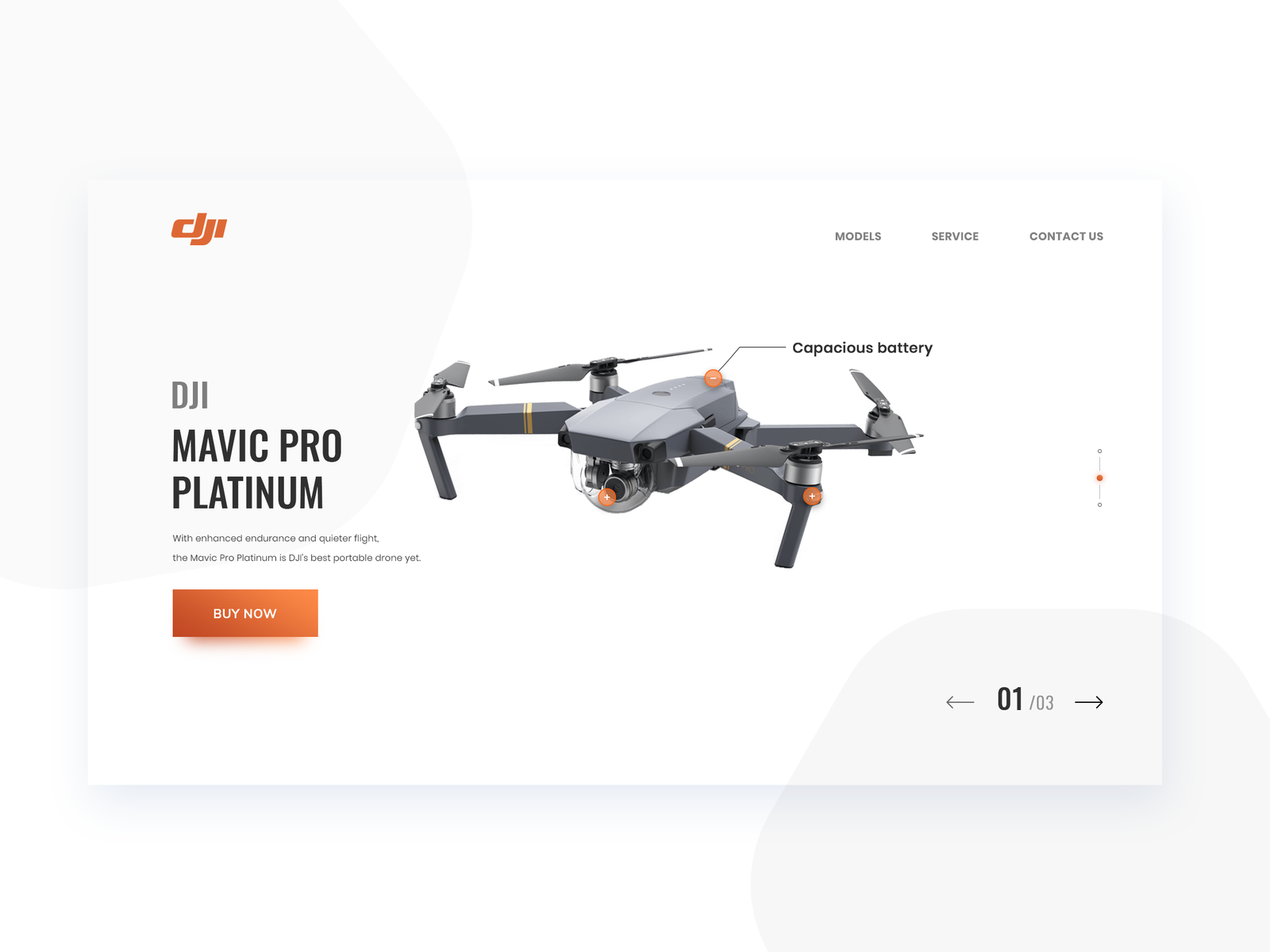The image showcases a sleek web page design with a minimalistic white background featuring subtle details. There are two faintly visible, irregular gray circles positioned in the upper left and lower right corners. These circles partially intrude upon a central white rectangular section, giving an impression of depth and layering.

In the upper left corner of the rectangle, the text "DJI" stands out in bright orange, while the upper right corner lists "Model", "Service", and "Contact Us" in subdued gray. Below this header, the brand name "DJI" reappears in gray, followed by the product name "Mavic Pro Platinum" prominently displayed in black. The accompanying description, "With enhanced endurance and quieter flight, the Mavic Pro Platinum is DJI's best portable drone yet.", provides a brief overview of the product's features.

An eye-catching orange button, centered below the description, invites immediate action with the bold, capitalized text "BUY NOW" in white.

In the lower right corner of the web page, navigational elements include a black arrow pointing left, a black arrow pointing right, and the text "01 / 03" in black and gray, indicating the current page in a series. The featured drone, mostly silver-gray with striking orange accents, is displayed prominently, highlighting its sleek and modern design.